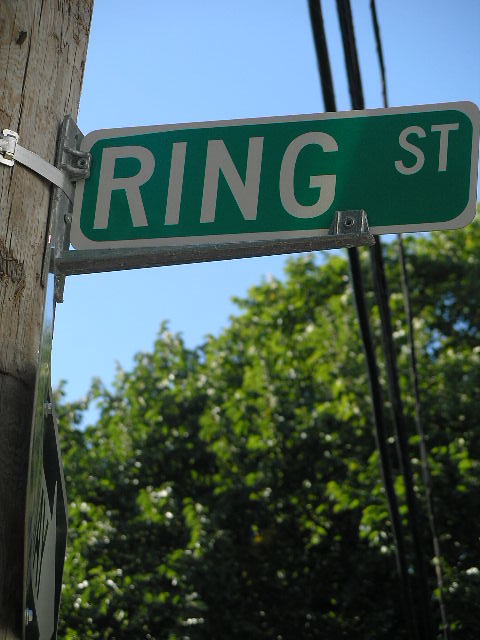This is a detailed, color photograph in portrait format featuring a street sign attached to a wooden telephone pole. The green rectangular street sign prominently displays the white capital letters "RING STREET." The sign is held high up on the pole with a sturdy metal anchor and an additional securing material. On the left side of the photograph, the telephone pole ascends vertically, and some black overhead wires run behind the sign. Another sign is visible peripherally, perpendicular to the main sign, with an arrow pointing to the right, indicating a one-way street. The bottom half of the image reveals a lush green tree, while the sky above is a bright, clear blue suggesting a sunny day.